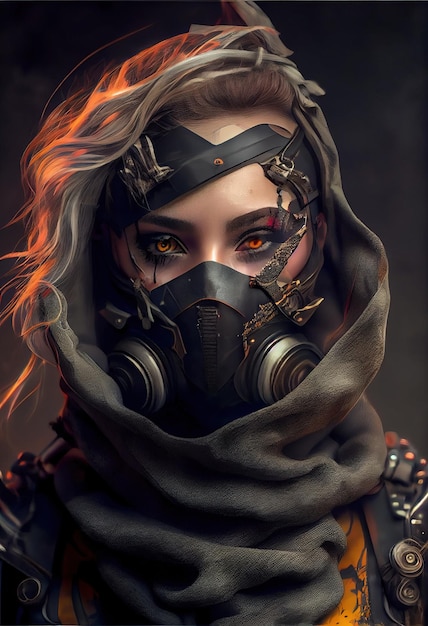This highly detailed color illustration portrays a woman, designed with realistic game graphics yet distinctly illustrated. She faces the viewer directly with striking orange eyes and thick eyebrows. Her long, silvery blonde hair flows to the left, partially wrapped in a cowl or shawl that covers her head and neck. The woman dons an intricate steampunk-inspired outfit, highlighted by a black respirator with silver caps and twin circular filters. The respirator, secured by numerous straps, covers her nose, leaving only her piercing eyes visible. Her elaborate uniform features leather straps with metallic buttons on her shoulders, hinting at complex mechanisms. The image is devoid of any additional elements or characters, focusing entirely on the confident and enigmatic woman.